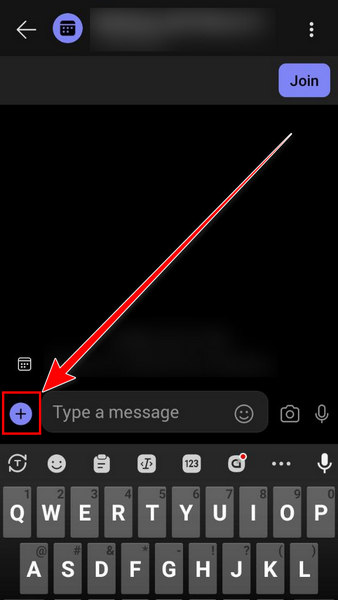This image is a screenshot from a smartphone application with a predominantly black background. At the top of the screen, on the left, a white back arrow icon is visible, followed by a purple circle containing a black keyboard icon. Adjacent to these, there's a text input box designated for typing messages, with three vertical dots (likely indicating more options) positioned on the far right.

Beneath this section, a medium gray bar spans across the screen, featuring a purple button labeled "Join." Further down, a prominent red arrow extends from the upper right corner towards the lower left, directing attention to a purple circle with a plus sign inside it. To the right of this circle is another input box labeled "Type a Message," flanked by a smiley emoji icon. Outside this box, on the far right, sit a camera icon followed by a microphone icon.

The lower portion of the screenshot displays a keyboard layout. The top row of this keyboard is dedicated to emojis, formatting options, numbers, and an additional microphone button. The subsequent rows show the first two lines of the QWERTY keyboard: the top line starts with 'Q' and ends with 'P,' while the second line starts with 'A' and ends with 'L.' The keys are medium gray with white lettering.